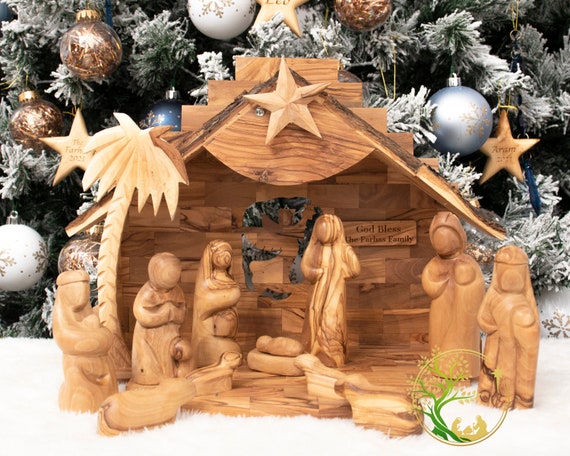This detailed image captures a beautifully hand-carved wooden nativity set, prominently displayed in front of a Christmas tree adorned with various festive ornaments. The nativity figurines, all made from light brown wood, include Mary and the baby Jesus in the manger, surrounded by wise men and animals, each showcasing meticulous craftsmanship. Above the wooden manger, a star sits atop, adding a touch of celestial charm. On the back wall of the manger, a sign reads, "God bless the Farless family," indicating the owners' name inscribed on it. The nativity scene also features a lighter palm tree on the left side, enhancing the scene's authenticity. 

In the background, a green evergreen Christmas tree, frosted with white snow, bursts with colorful ornaments including white, brown, and blue bulbs, alongside various hanging stars. A decorative circle bearing a tree of life is visible at the bottom right corner of the image. Additionally, a pair of figures, possibly a man and a woman, seem to be bending over something in the far corner, though their specific activity remains unclear. This scene intertwines the reverence of the nativity with the festive spirit of Christmas.